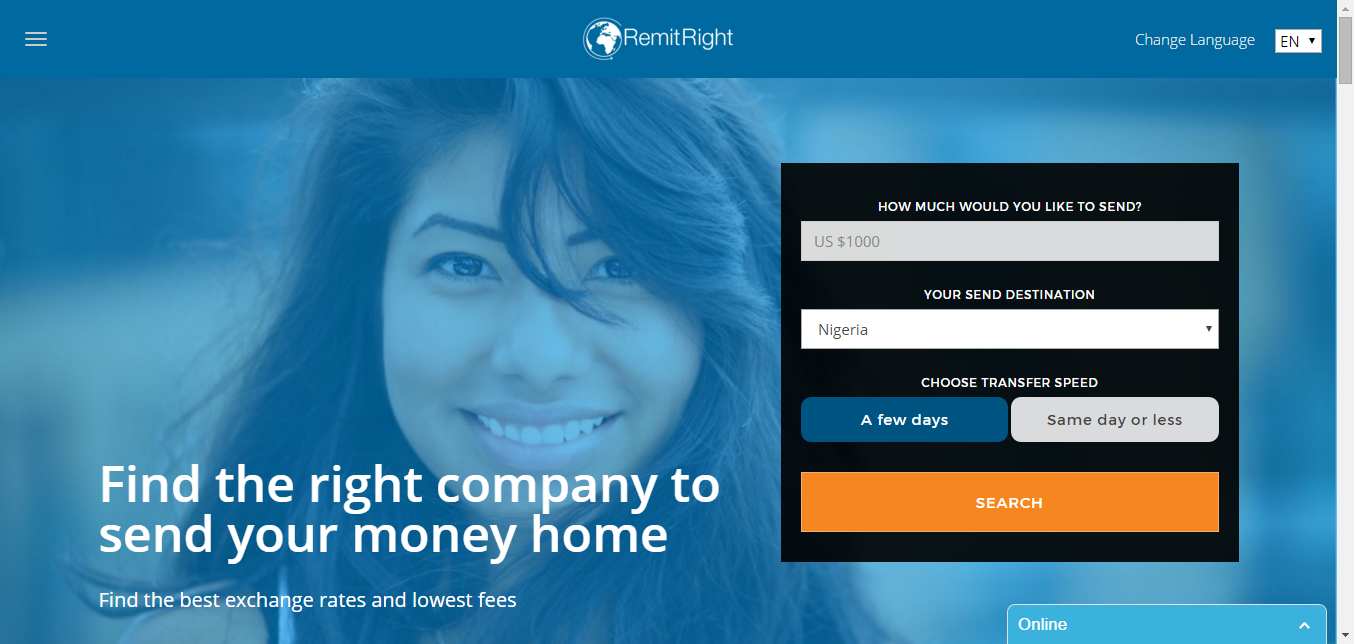The screenshot depicts a webpage from "Remit Right," prominently featuring the logo with text and a globe icon centered on a blue bar at the top. On the left side of this bar is a hamburger menu, while the right side displays a "Change Language" option with English (EN) currently selected. 

The central focus of the image is a young woman, likely in her mid-20s with potentially Hispanic features and dark brown hair, facing the camera. She is overlaid with a blue gradient at approximately 50% transparency. Beneath her face, white text reads: "Find the Right Company to Send Your Money Home. Find the Best Exchange Rates and Lower Fees."

To the right of the woman, a black box contains input fields. The first field, labeled "How much would you like to send?", defaults to USD $1,000. Following this, there is a "Send to your destination" field, pre-set to Nigeria. Below that, options for transfer speed are presented: a blue button for "A Few Days," a white button for "Same Day or Less," and an orange and white button labeled "Search."

In the bottom right corner of the screen, a light blue tab with an upward arrow and the text "Online" is displayed, suggesting it may be a clickable feature for customer support, either through a chat representative or a bot. The tab remains at the bottom of the screen, indicating its availability for questions or assistance.